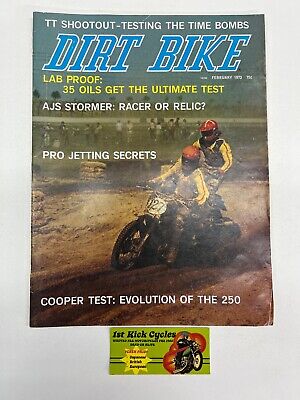The image is of a **Dirt Bike** magazine cover, dated February (year unclear). Dominating the cover is an action shot of two men on a dirt bike, emblazoned with the number 127, riding on a dirt track. Both riders are dressed in yellow jackets with red stripes down the sleeves and wearing red helmets. The scene is set against a backdrop where the dirt is distinctly brown, and a muted crowd watches the race. 

At the top of the cover, in white text, it announces “**TT Shootout: Testing the Time Bombs**.” Below, in yellow, it reads “**Lab Proof: 35 Oils Get the Ultimate Test**.” The main title "Dirt Bike" is prominently displayed in large blue letters, trimmed with white. Further down, in white text, it features articles titled “**AJ Stormer: Racer or Relic**,” and “**Pro Jetting Secrets**.” Near the bottom, another key highlight reads “**Cooper Test: Evolution of the 250**.” Additionally, at the bottom of the cover, there is a green business card with “**First Kick Cycles**.”